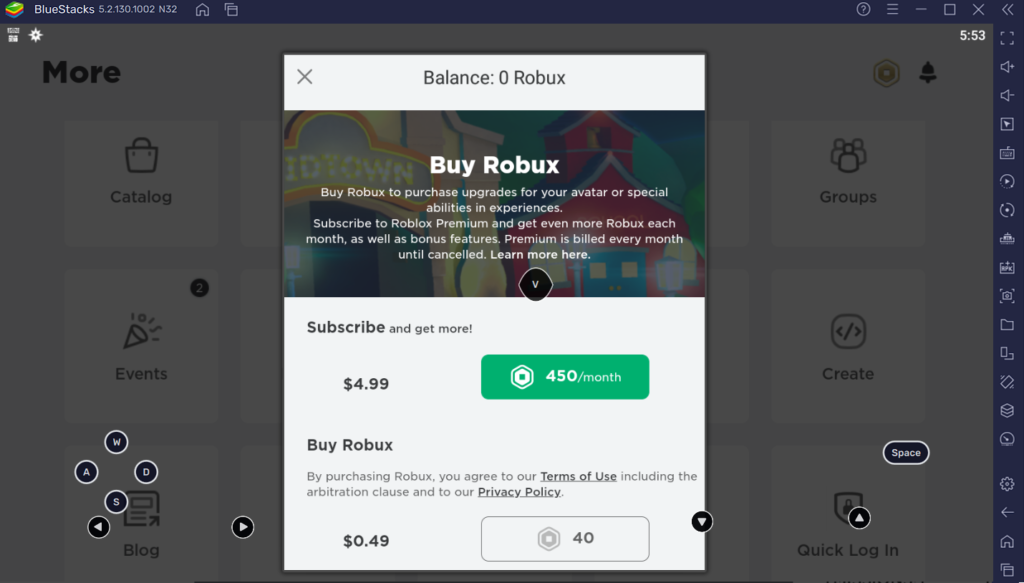A detailed screenshot of the BlueStacks app is displayed. At the top of the image, a thin navy box encapsulates the BlueStacks logo along with a string of alphanumeric characters. Adjacent to this, there are colorful icons in green, red, and blue. The navigation panel features a series of icons including a house, paper documents, a question mark in a circle, lines, a box, an 'X' symbol, another box, volume controls, a badge-like icon, circles, paper stacks, squares, a folder, a phone, additional papers, a cogwheel, an arrow, a house, and others. The time displayed in the corner reads 5:53.

The main interface presents a white and gray background with multiple white squares, each designated with black text and small icons. Categories include 'Catalog' marked by a shopping bag icon, 'Groups' with people icons, 'Events' represented by a funfetti icon, and 'Create' and 'Blog' sections indicated by corresponding icons. Near the blog section, navy circles with white letters A, W, D, and S are visible alongside two black circles with white arrows.

The header 'Quick Login' features a shield icon. Below, a navy box labeled 'Space' is displayed. Overlaid on this interface is a white pop-up window indicating "Balance: 0 Robux" against a backdrop featuring red and white buildings.

The pop-up prompts users to buy Robux with a message that reads, "Buy Robux to purchase upgrades for your avatar or special abilities and experiences. Subscribe to Roblox Premium and get even more Robux each month, as well as bonus features. Premium is billed every month until canceled. Learn more here." A black circle with a white 'V' is present.

At the bottom, a white background with black text invites users to "Subscribe and get more for $4.99." Adjacent to this, a green box with white text reads "$450 a month" followed by a circular icon. Additional text emphasizes, "Buy Robux. By purchasing Robux, you agree to our terms of use, including the arbitration clause and privacy policy," with a cost listed as "$0.49." A nearby white box displays "$40" alongside the circular icon again.